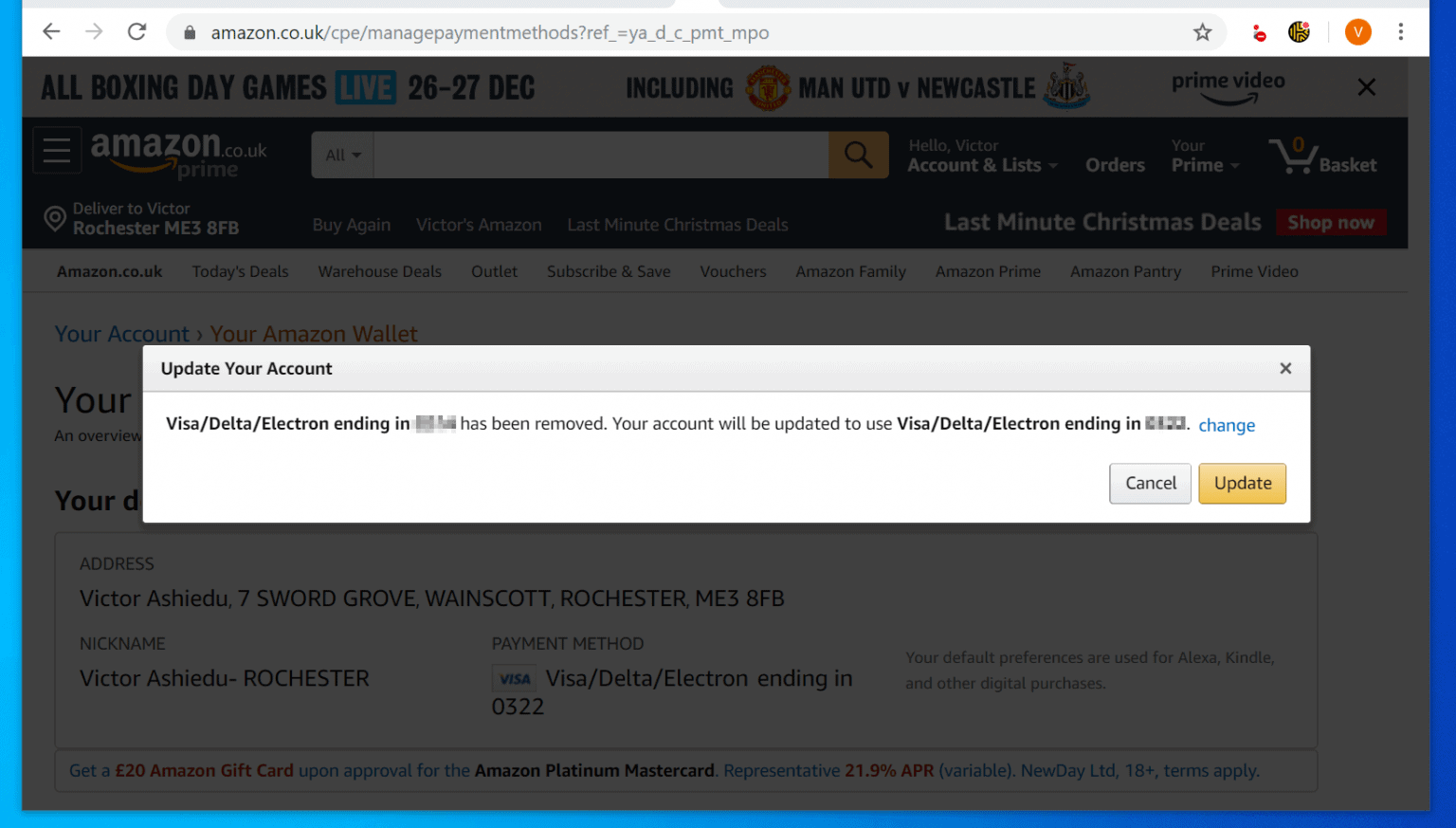A detailed screenshot from the UK version of Amazon (Amazon.co.uk) is displayed, specifically from the "Manage Payment Methods" section of the webpage. The focal point of the screenshot is a dialog box with a prominent grey bar at the top left, titled "Update Your Account." Beneath this heading, in bold text, it reads "Visa/Delta/Electron ending in [number pixelated] has been removed." Following this, there is a notification indicating that "Your account will be updated to use Visa," with the same bold text format. It then repeats "Visa/Delta/Electron ending in [number pixelated]" to denote the updated payment method. The sensitive number details have been pixelated to maintain privacy.